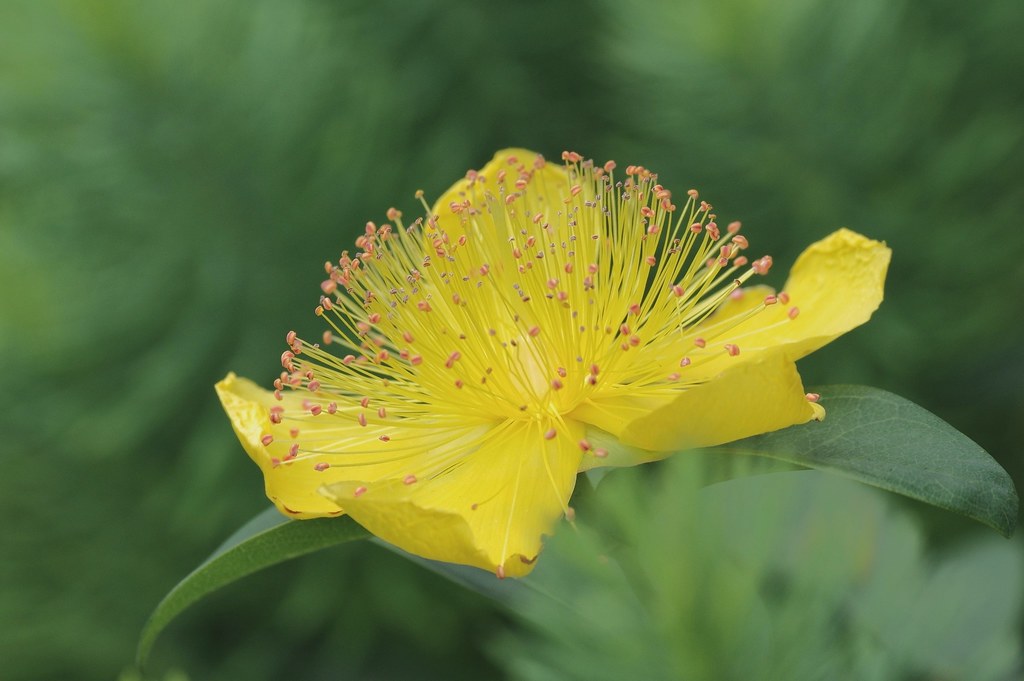A close-up of a vibrant, yellow Hypericum flower is showcased in this detailed photograph. The flower, which grows on a small plant, features five broad petals that curve slightly upwards at the edges and have a delicate, exotic appearance. Emerging from the flower's center are numerous, slender stamens with pink-tipped filaments, bearing seeds or pollen. The flower is set against a backdrop of deep green foliage, which is beautifully blurred to highlight the sharp, intricate details of the blossom. The leaves, found on either side of the flower, are long and broad with angled veins curving down the center. The overall deep green background suggests a lush, floral setting, enhancing the striking contrast and beauty of the yellow flower.